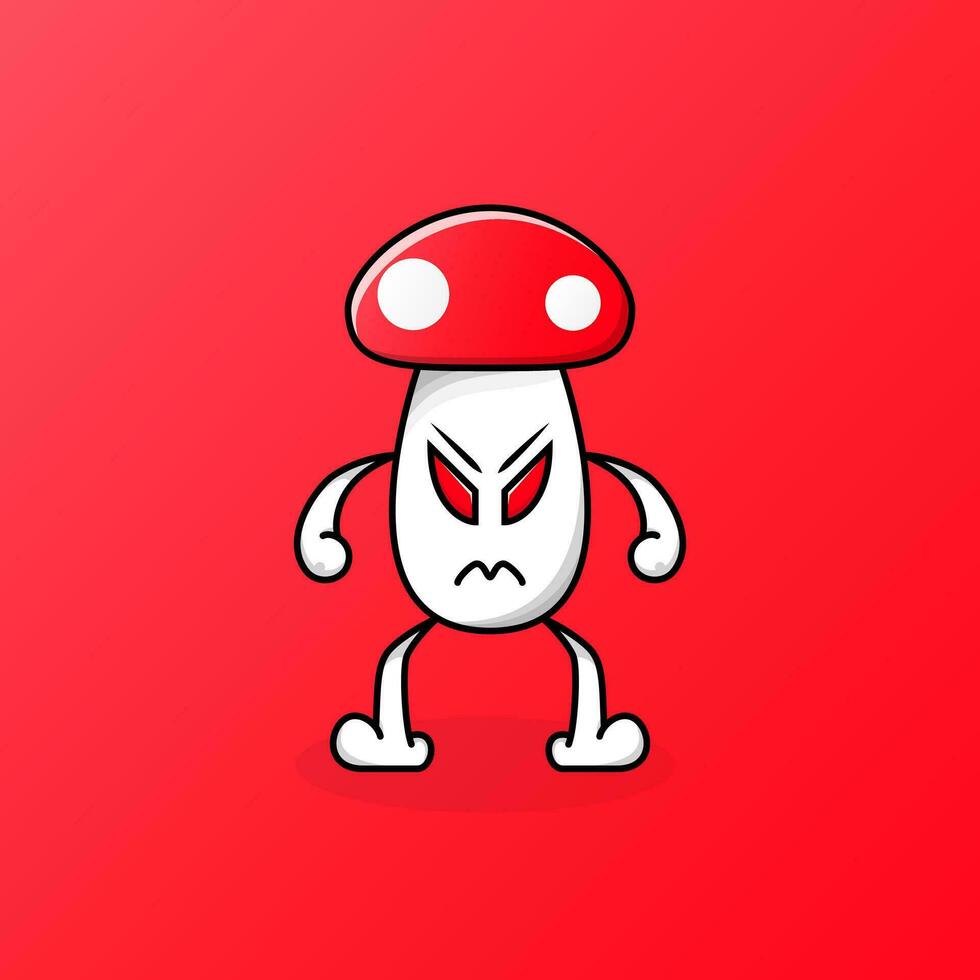The image depicts a cartoon character resembling an angry mushroom, set against a solid cherry red background. The character features a red mushroom cap with two prominent white circles, topping a bean-shaped white body. Its facial expressions include menacing, slanted red eyes, and eyebrows angled sharply towards its nose, enhancing its angry demeanor. The mouth is a squiggly line shaped like an 'M,' further emphasizing the character's malevolent expression. The mushroom figure has two arms, shaped like upside-down commas, and stands in a cowboy-like pose with its stubby white legs, adding a touch of humor to its angry appearance. The overall design suggests it could be a whimsical antagonist in a video game or a children's book.